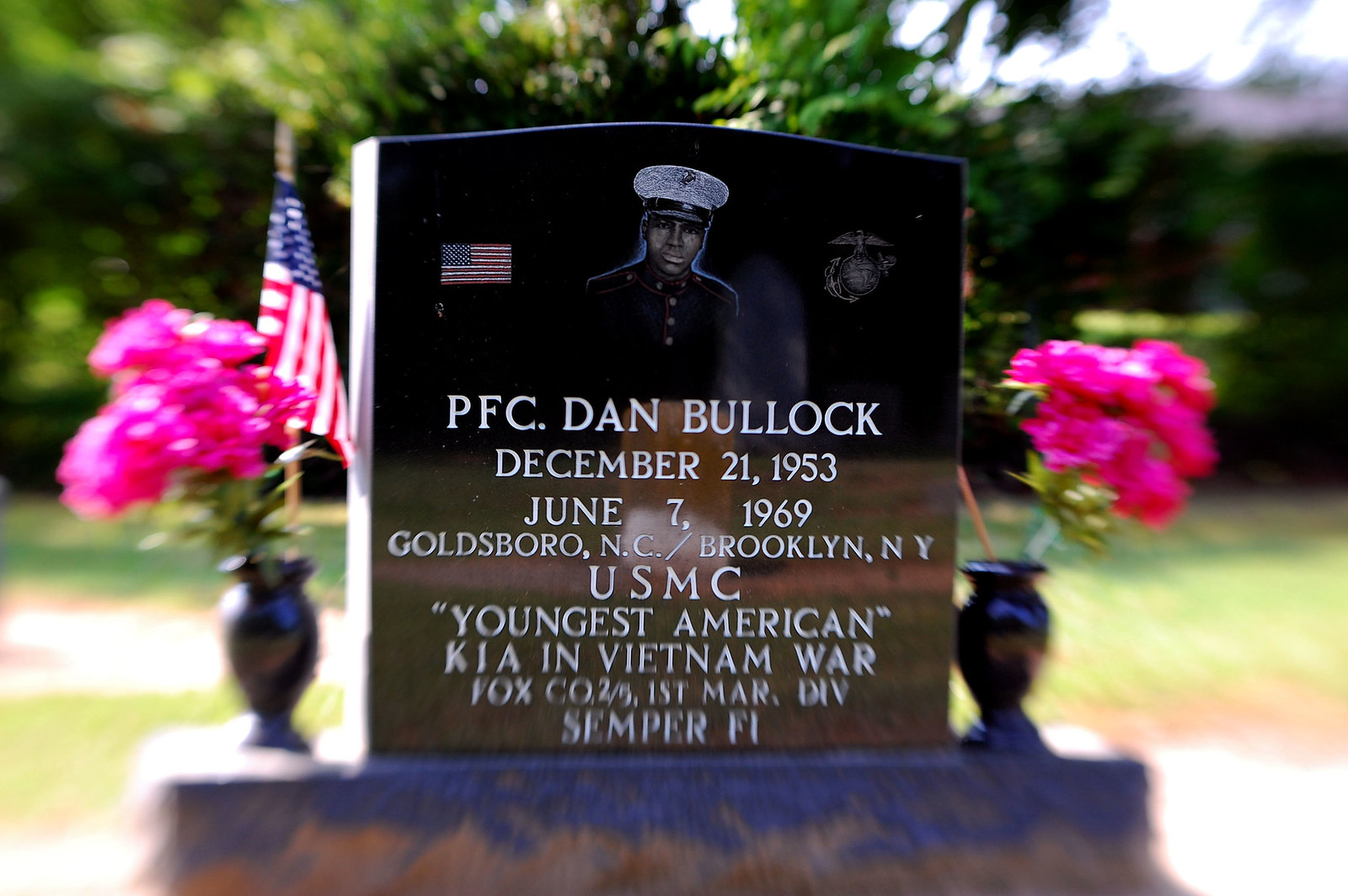The image captures a solemn scene of a soldier's grave, blurred into a serene background of trees and greenery. At its center stands a black gravestone featuring a photograph of PFC Dan Bullock, an African American soldier dressed in a uniform with a white hat. Inscribed in white text are the details: "PFC Dan Bullock, December 21, 1953 - June 7, 1969, Goldsboro, North Carolina / Brooklyn, New York, USMC, youngest American KIA in Vietnam War, Fox Co, 2/5, 1st Marine Division, Semper Fi." Flanking the gravestone are two black urns or vases, each containing five or six pink roses. The left vase also holds a small American flag, while another flag is draped iconically to the left of the gravestone. The right side features a circular symbol with a falcon. The scene is a poignant tribute, emphasizing honor and remembrance.